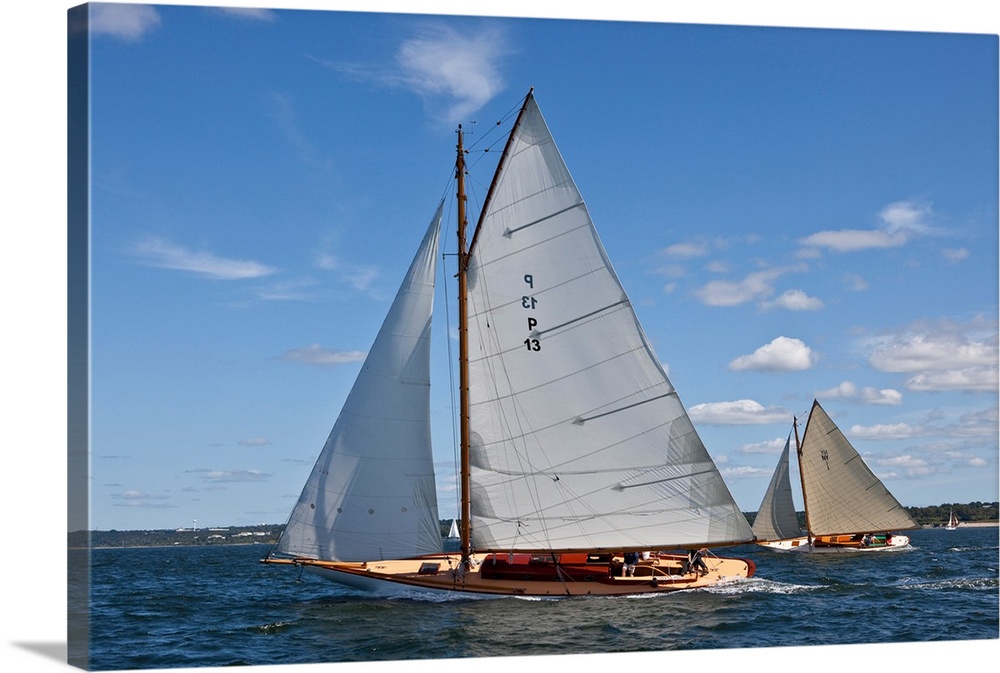In this rectangular canvas print, measuring approximately five inches wide and three inches high, the scene portrays a serene outdoor setting on a large lake under a blue sky with scattered white and gray clouds, notably condensed over the lower right side. Two nearly identical, long and narrow sailboats glide across the vibrant blue water, creating gentle waves with a bit of foam trailing behind. Each boat, featuring a dark wooden hull, is manned by a single person handling the sails and rudder. The larger sail is positioned towards the back, while a smaller sail is mounted at the front. On the left side of the image, a thin strip of land reveals buildings, and on the right, lush trees and possibly another sailboat near a beach area. The picture captures the peacefulness of a day spent sailing, framed against the backdrop of distant land with houses and trees.